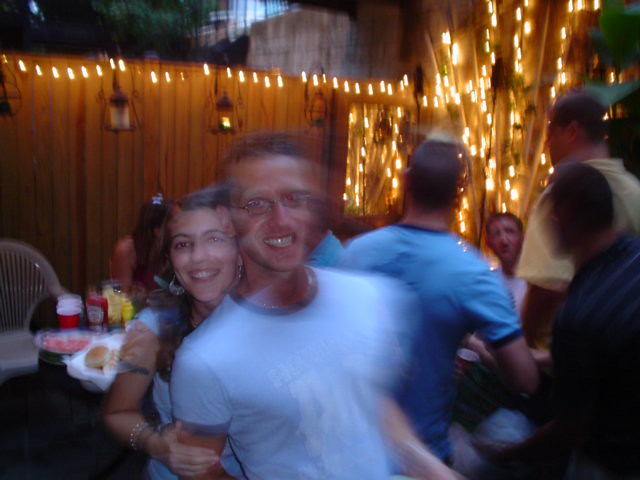In this blurred image, it appears to capture an outdoor party in someone’s yard. A prominent wooden fence adorned with twinkly string lights stretches across the background, featuring small lanterns or candles—though only one light is visibly lit amidst the array. To the right, strings of lights possibly illuminate a nearby tree. A mysterious, well-lit box on the fence resembles a mirror but remains indistinct due to the blurriness.

In the foreground, a man and a girl stand together; the girl is behind the man, holding his upper arms. The man wears a light-colored T-shirt with darker trim at the collar, has brown hair, glasses, and a smile on his face. The girl, also smiling, has dark hair draped over her right shoulder and is adorned with multiple bracelets. Her hand rests on the man’s right upper arm.

The background reveals a table set with ketchup, mustard, red solo cups, and plates of food, indicating a festive atmosphere. Additionally, the image shows people further back, with one person’s back visible as they sit, seemingly part of a circle of attendees. The overall scene, despite the blur, emanates a sense of warm, lively celebration.